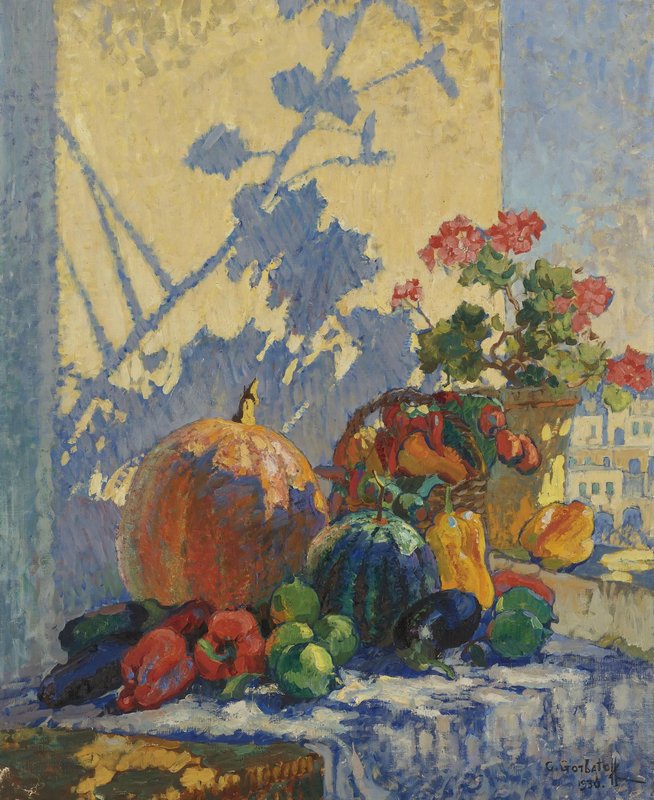The image is an impressionistic still life situated on an open porch. It showcases a table adorned with a blue and white tablecloth that has a signature of an artist dated to 1930, though the artist's identity is unclear. The scene captures a variety of vegetables including pumpkins, squashes, tomatoes, eggplants, peppers, and possibly some limes, arranged in a pleasing display. Next to these, pink and red geraniums are potted in a larger pot, resting on the ledge of the balcony. The flowers cast distinct blue shadows on a nearby wall, highlighting the intricate interplay of light and color. Beyond the balcony, several old-world style buildings stretch out into the distance under a blue sky dotted with clouds. The image merges natural elements with an urban backdrop, blending still life with a vibrant outdoor setting.